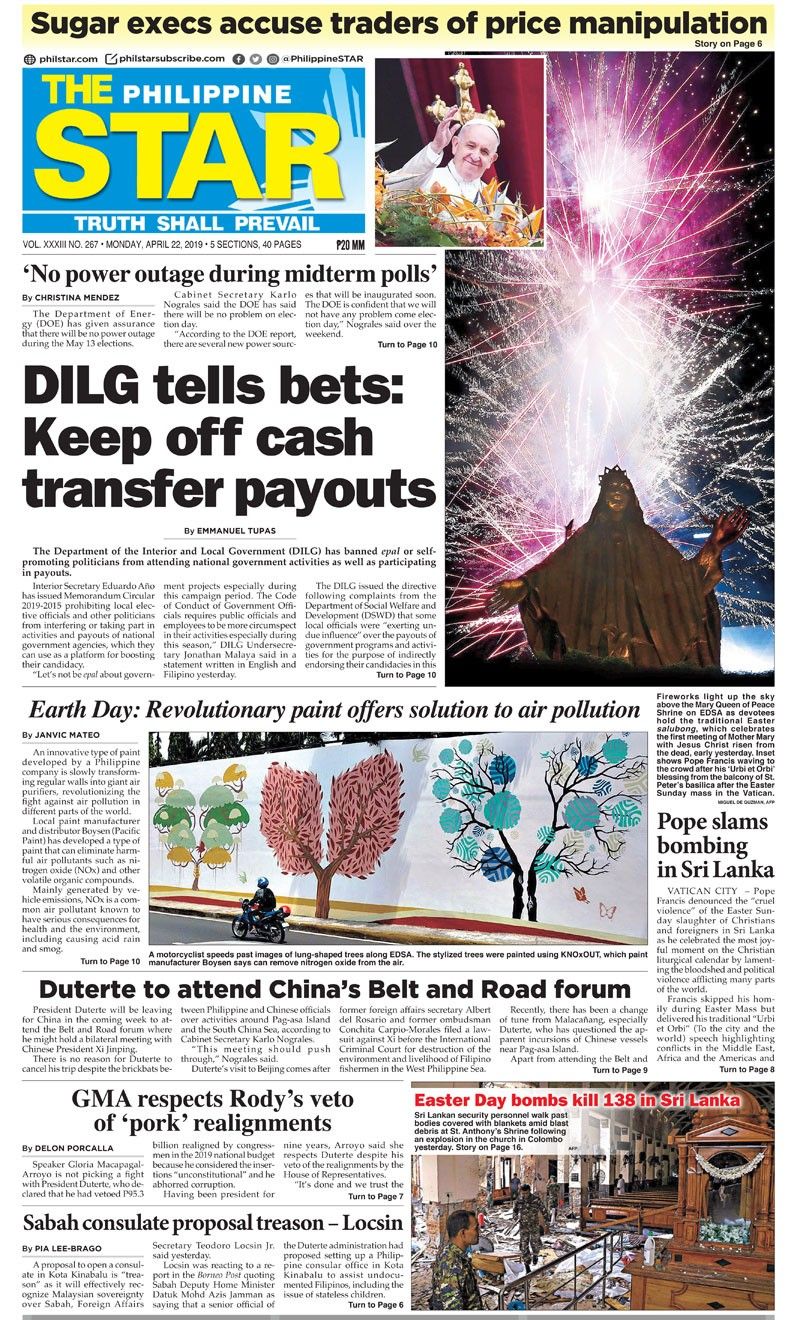The newspaper front page features a vivid yellow header that transitions smoothly into white towards the bottom. Prominently displayed in large black text at the top is the headline, "Sugar Execs Accuse Trader of Price Manipulation," with a smaller note below it on the right stating, "Story on Page 6". 

Moving down to the left side, there's a blue background adorned with a white snowflake or star icon positioned on the right. Superimposed on this background, the text transitions from yellow to white: "The" in yellow, "Philippine" in white, and finally "Star" in bold yellow text. Beneath these words, separated by a thin white line, is the newspaper's slogan in white text: "Truth Shall Prevail."

To the right, an evocative photograph depicts St. Francis blessing a bed of flowers with his right hand, set against a backdrop of a gold cross and a luxurious red velvet curtain.

Further down on the right, a vertical image with a stark black background showcases an array of white and pink fireworks extending across the height of the image. At the base is a grand brass or gold statue of a figure draped in a shawl, standing with one arm extended to the left and the other to the right.

On the left side, an article titled "DILG Tells Bets Keep Off Cash Transfer Payouts" by Emmanuel Tupas is prominently featured. Below this article, another titled in italics, "Earth Day: Revolutionary Paint Offers Solution to Air Pollution," adds to the diversity of topics covered on the front page.